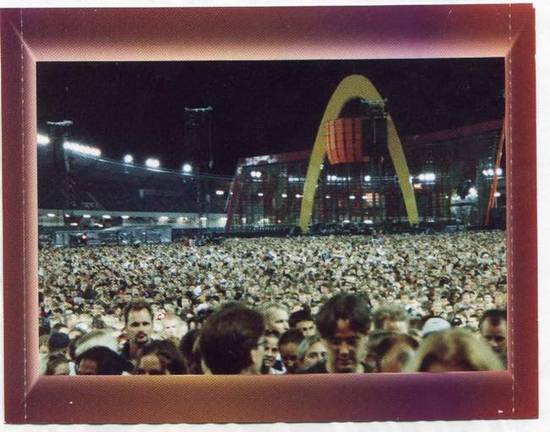The photograph captures a large nighttime assembly of mostly young people, likely in their late teens to early twenties, congregated in what appears to be a stadium. The sky is pitch black, contrasting with the bright stadium lights that illuminate the scene. The image is notably framed by a distinct red, pink, yellow, and purple border, which suggests that it might be a snapshot of a broadcast or simply an artistically framed photograph.

In the background, a prominent golden arch stands out, accompanied by an orange object in front of it, adding a focal point to the scene. There's a red-topped wall with writing on it and a structure that resembles a stage or possibly part of the stadium's architecture, where glass elements and small windows are visible. This structure is set against a backdrop of tiered stadium seating, filled with more attendees. The overall ambiance and the scale of the crowd, which could easily number in the hundreds or thousands, hint at a significant event, potentially a concert or a sporting event, though the exact nature remains unspecified.